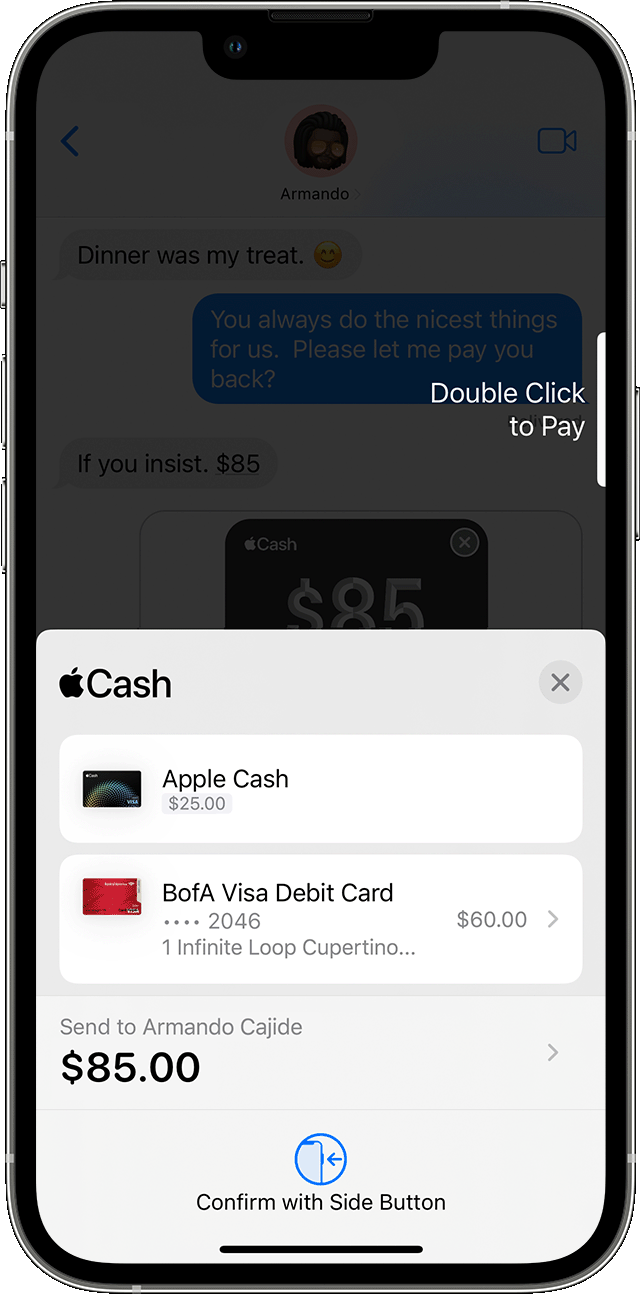The image features a silver smartphone with a slightly bezel-rounded rectangular shape, displayed against a solid white background, making it appear as though it's floating in an empty void. The smartphone's right edge houses a long rectangular button, while the left side contains three buttons: two of equal length and a smaller, presumably power button, at the top. 

On the screen, a chat window appears grayed out, showcasing a series of messages. The first message reads, "Dinner was my treat." This is followed by a response saying, "You always do the nicest things for us, please let me pay you back." The final message states, "If you insist, $85." Overlaying this conversation, the active payment interface of the Apple Cash app is prominently displayed, ready to facilitate the transaction.